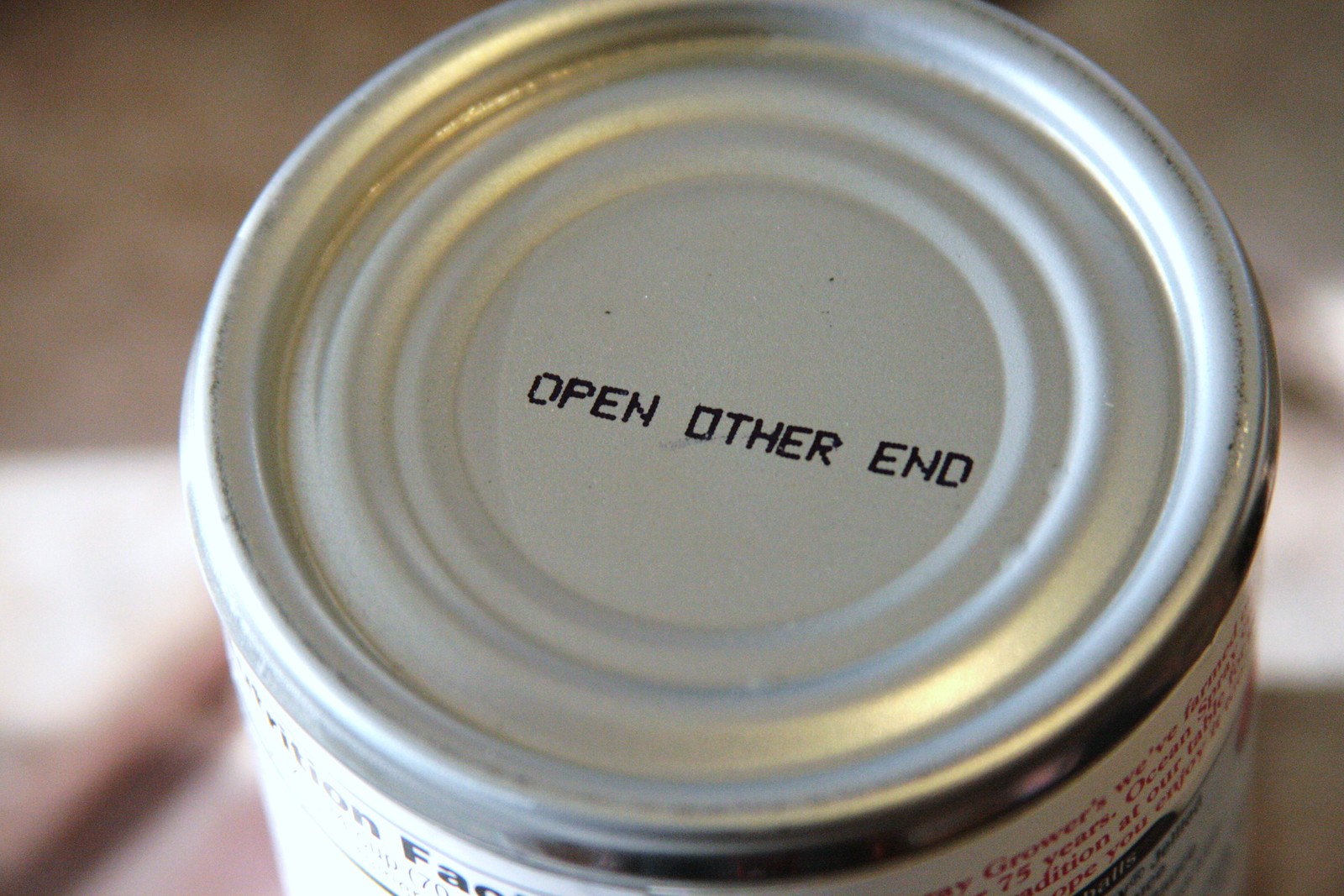The image depicts a close-up view of the metallic bottom of a can, with the circular surface taking up most of the frame. Prominently displayed in black capital letters at the center of the bottom are the words "OPEN OTHER END". The shininess of the metallic surface reflects light, giving the impression of natural lighting, possibly from a nearby window. The bottom left edge of the can features a part of a white label with the words "NUTRITION FACTS" visible in black letters, although the rest of the label is cut off and unreadable. On the right side of the can, in red lettering, the word "GROWERS" is observed, along with "75 years." This minimal information, coupled with the indistinct product details, suggests it might be a food product, potentially something like tuna, inferred from another partially visible word, "ocean," near the red lettering. The can is placed against a background that appears to be a light-colored table, possibly white or beige, with a small, out-of-focus area that might be a cloth bunched up on the left. The overall emphasis is on the clean, metallic bottom of the can, underscored by the helpful instruction to "OPEN OTHER END."